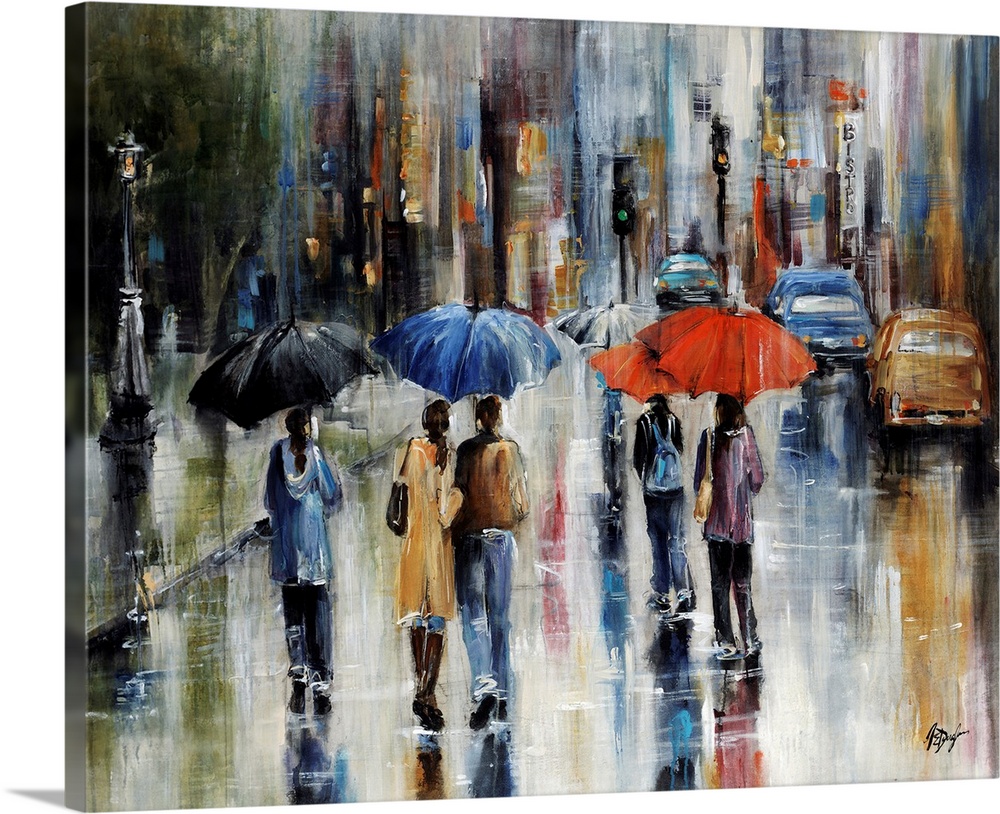The painting depicts a bustling city street on a rainy day, where at least six people with umbrellas are walking along a wet sidewalk. The street glistens with the reflections of watercolors blending together, giving a rain-soaked, impressionistic feel to the scene. Vibrant umbrellas in black, blue, red, gray, and black-and-white patterns provide pops of color against the washed-out, indistinct backdrop. In the background, there are multiple cars in hues of teal blue, dark blue, and brown, positioned along the street. A traffic light and a street lamp are visible, contributing to the urban landscape. A distant green tree and a sign saying "Bistro" add to the city ambiance. The figures are dressed in casual attire, with some carrying purses and backpacks. The artwork's signature sits in the lower right corner, though it remains illegible.